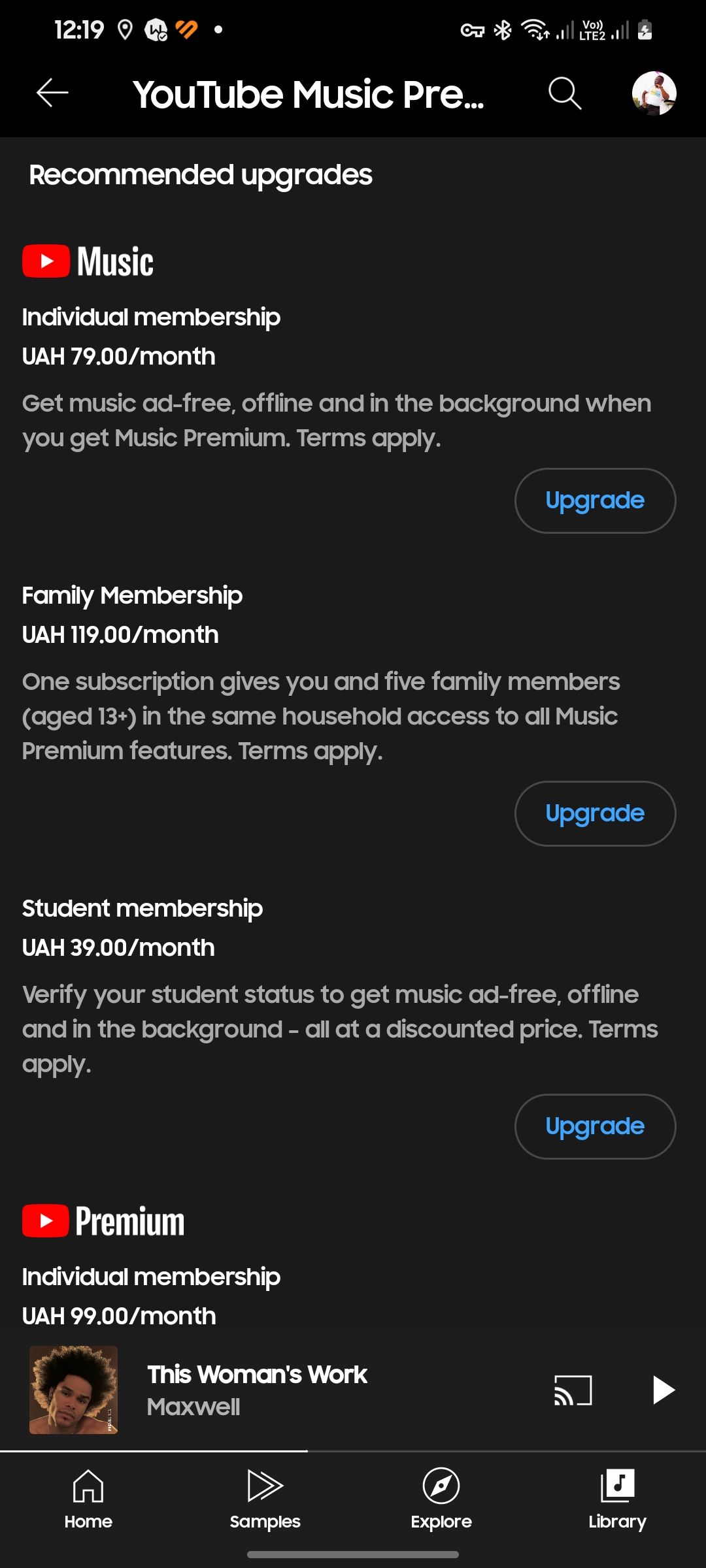The image is a screenshot with a completely black background. In the upper left corner, the time is displayed as 12:19. In the upper right corner, there is a battery icon that shows approximately half charge.

Beneath this, there is a navigation row featuring a back arrow, the "YouTube Music" title followed by an ellipsis ("..."), a search icon, and a user's avatar depicting a person with dark skin wearing a white t-shirt. The gender of the individual in the avatar is not clear.

The next row is labeled "Recommended Upgrades." Below this, there is a promotion for "YouTube Music Individual Membership" priced at UAH 79 per month, offering benefits such as ad-free music, offline access, and "Music Premium" features, with terms and conditions applied. There is a light blue button labeled "Upgrade."

Following this, there is an option for a "Family Membership" at UAH 119 per month, which provides the same "Music Premium" benefits for the subscriber and up to five family members aged 13 or older within the same household, with similar terms. This also includes a light blue "Upgrade" button.

Next, an option for "Student Membership" is offered at UAH 39 per month, which requires verification of student status. This membership delivers ad-free music, offline access, and other benefits at a discounted price, accompanied by a light blue "Upgrade" button.

Further down, there is a "YouTube Premium Individual Membership" available for UAH 99 per month.

At the bottom of the screenshot, a song titled "This Woman's Work" by Maxwell is currently playing. The navigation bar at the bottom displays options for "Home," "Samples," "Explore," and "Music Library."